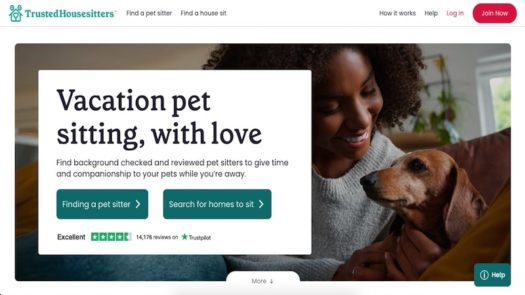This screenshot from a webpage showcases a comprehensive layout with a focus on pet sitting services. At the top, there is a white rectangular banner featuring a gray icon resembling a dog house with ears. Next to the icon, in gray font, it reads, "Trusted House Sitters™." Alongside this text, navigation options in black font include: "Find a Pet Sitter," "Find a House Sit," "How It Works," "Help," and "Log In." A prominent red button labeled "Join Now" is also visible.

Below the banner is a heartwarming photograph of a smiling Black woman with natural hair, wearing a gray crewneck sweater. She is tenderly holding a brown dachshund, whose muzzle shows signs of graying, indicative of his senior age. The dachshund appears content, with his left profile and brown eyes directed towards the left, all while the woman beams down at him with her very white teeth.

Overlaying the left side of the photo, a white square contains black text: "Vacation pet sitting, with love. Find a background checked and reviewed pet sitter to give time and companionship to your pets while you're away." Below this message are two gray buttons with white font: on the left, "Finding a Pet Sitter," and on the right, "Search for Homes to Sit."